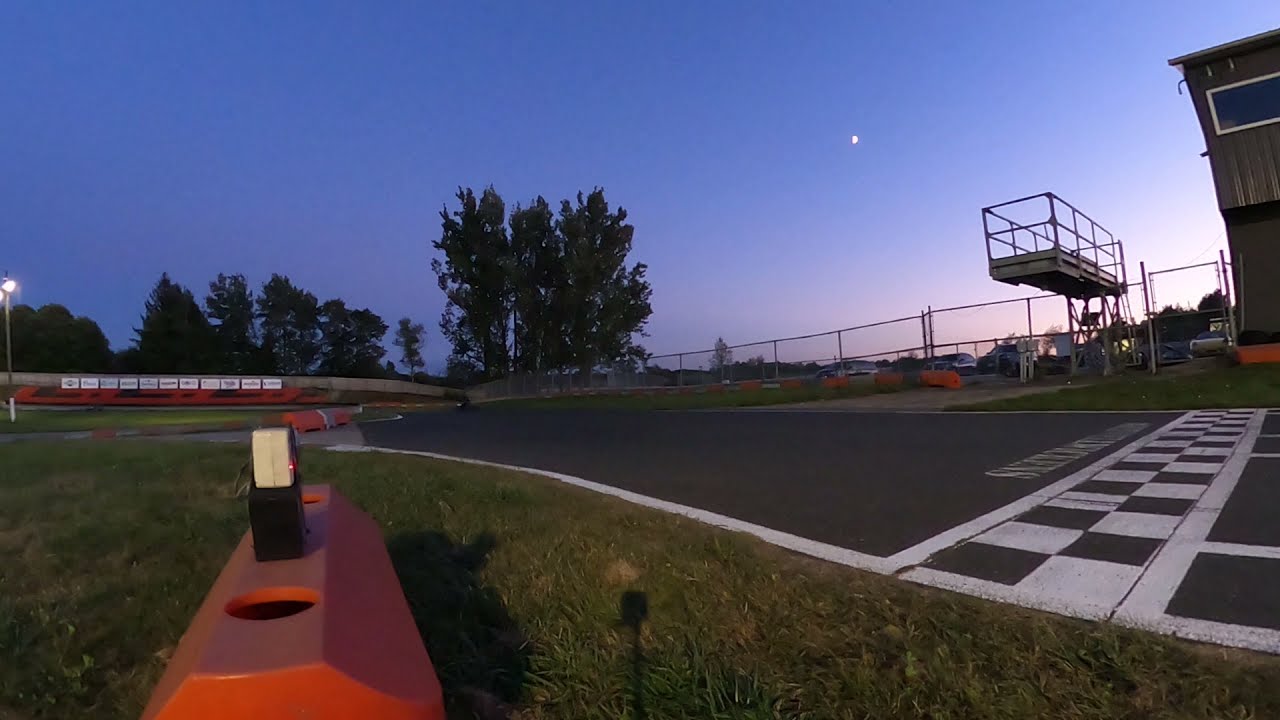The image depicts an athletic racetrack, likely photographed from the center grass area near the checkered start/finish line, which is situated at the bottom right corner. The track is bordered by white lines and surrounded by a backer board with advertisements on the far edge. The sky above transitions from a deep blue into a lighter hue, suggesting the time is either dawn or dusk, with the sun below the horizon and the faint moon visible. The landscape beyond the track includes a grove of large trees and a parking lot with cars. In the foreground on the bottom left, there are orange objects, possibly track equipment, scattered on the grass. The right side of the image features a brown building with large, tinted windows, likely housing record keepers or coaches, alongside an observation platform with a ladder. Additional lighting fixtures are still illuminated around the track, emphasizing the dimly lit, serene ambiance of the scene.